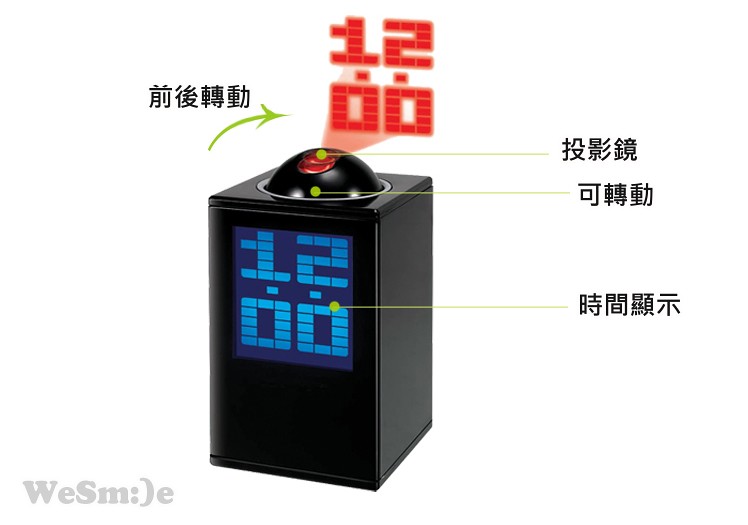This is a detailed, color illustration featuring a tall, slender, black rectangular 3D object, possibly a projector, set against a white background. The object has a black semi-circular dome on top, which appears to function as a rolling control. There is a small red circle in the center of this dome. The front of the rectangular object features a display screen with a dark blue background, displaying the time "12:00" in a segmented digital format using small square blocks. Above the black dome, the numbers "12:00" are also projected in red with a subtle pinkish-grey lighting effect underneath, mimicking a wall projection. There are various elements of oriental or Asian writing positioned near the object, including to the left and right, with green arrows pointing towards the writing and different parts of the object. Additionally, in the bottom left-hand corner, there is a greyscale watermark that reads "W-E-S-M; (E)" stylized to resemble the phrase "We Smile" in a playful manner.